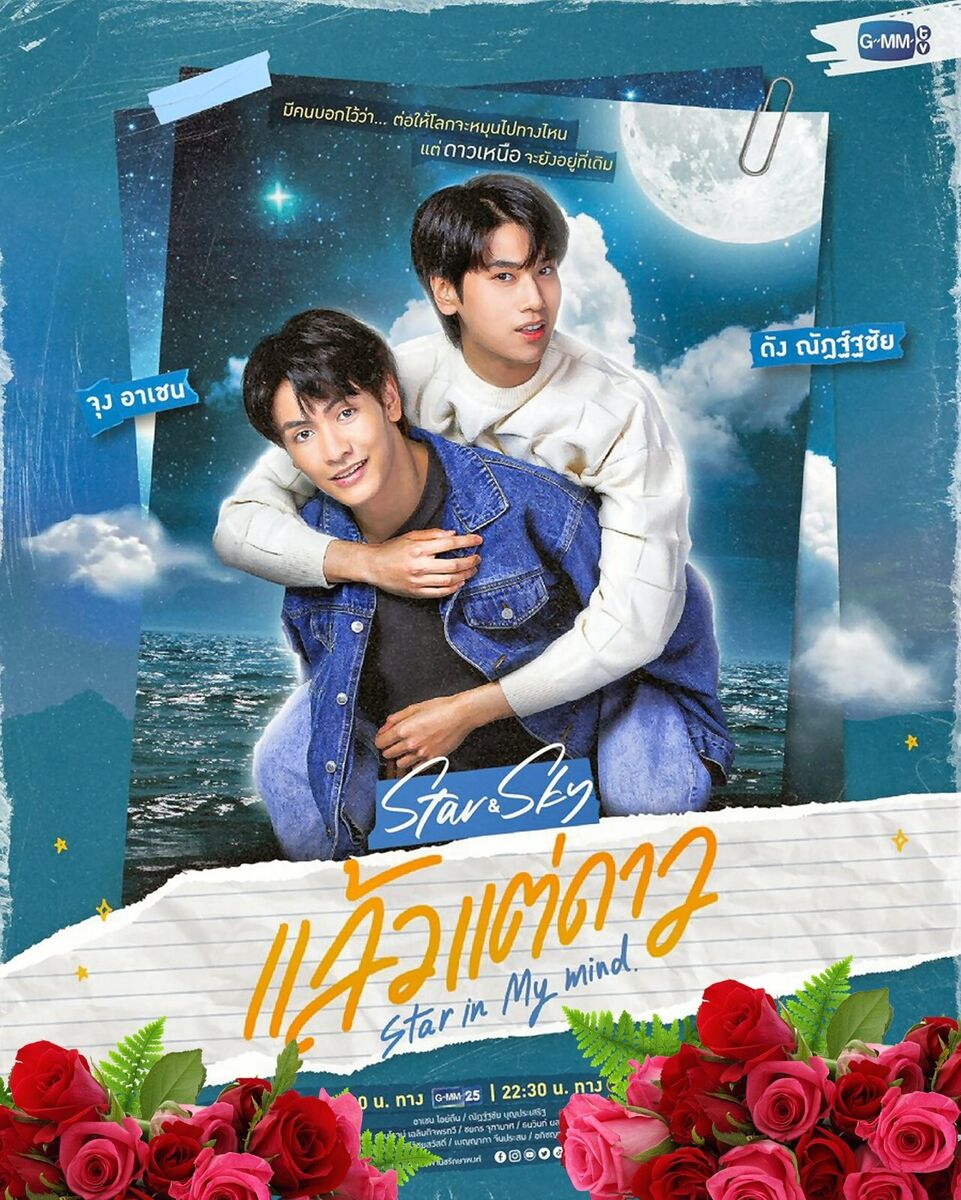The image is a detailed and vivid poster, featuring two dark-haired Asian men at its center. The background transitions from a serene ocean at the bottom to a night sky adorned with a moon, stars, and a few wispy clouds. Surrounding the image is blue paint with a few mountains peeking in.

In the upper right corner, the initials "GMM" are prominently displayed. The man in the foreground, wearing a black t-shirt under a denim jacket, carries the second man piggyback. The man riding piggyback is clad in a white long-sleeved sweater, paired with blue denim pants, and has a playful expression on his face. They both share a moment of lightheartedness, with the one in the denim jacket smiling lightly.

Beneath them is a torn piece of notebook paper stretching from left to right, with the title "Star In My Mind" written in orange. Below this, in white font, are the words "Star & Sky," which appear again in blue text. The sides of the poster feature additional script writing in an Asian language.

In the lower right and left corners, lush red-pink roses with green ferns add a touch of natural beauty. The bottom section also contains dates, specifically "22 through 30," amidst other script elements. There are visible tape marks and a paper clip indicating it has been fastened in some manner. The entire scene projects a blend of digital art and photography, promoting an Asian movie or television show with its blend of imagery and text.